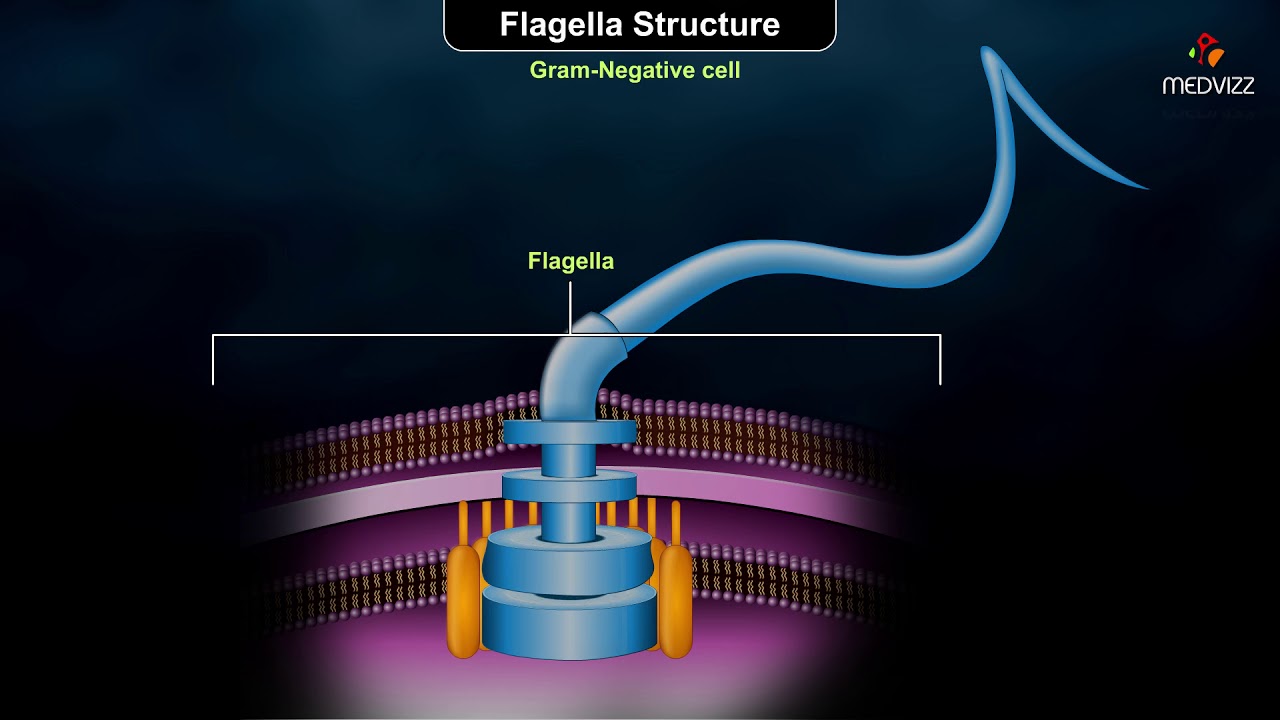The graphic titled "Flagella Structure" depicts the anatomy of a flagellum within a gram-negative cell, highlighting a detailed scientific illustration. Centered in the image, the title "Flagella Structure" appears at the top in white font on a black background, with "Gram Negative Cell" directly beneath it in light green. To the top right is the MedViz logo, composed of green, red, and orange colors, accompanied by the text "MEDVIZ".

The main illustration features a complex cross-section of a cell. A conspicuous blue structure, representing the core, is encircled by several orange sacs and flanked by small, purple layers that suggest the cell envelope or membranes. A long, rope-like appendage, labeled "Flagella," extends from the core structure and curves gracefully to the top right of the image. This flagellum is highlighted by a green label and a white bracket, underscoring its length and position. The background of the image is primarily black with subtle lighter shades, enhancing the contrast and visibility of the elements within the diagram.